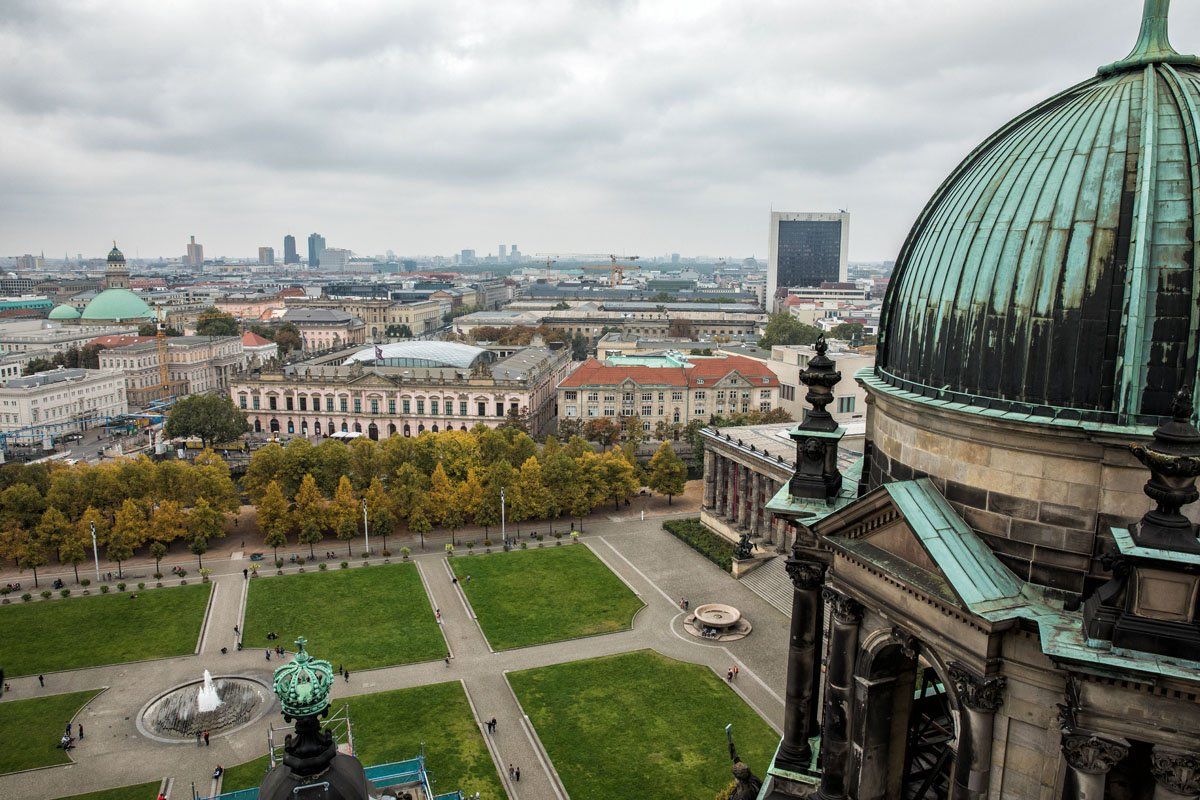The image captures a bird's eye view from atop a tall building, showcasing a sprawling cityscape that seamlessly blends ancient and modern architecture. Prominently, an aged copper green dome, adorned with patches of black likely due to moss or mold, stands out against the city's skyline. Below, meticulously manicured square patches of green grass are interspersed with walkways, creating a grid-like pattern. In the center of this greenery, a water fountain shoots a stream of water high into the air. A line of carefully trimmed trees, hinting at the onset of fall with their changing colors, adds a natural element to the urban setting. Beyond this foreground, the city extends into the distance, featuring a mix of old buildings with elegant domes and modern structures. The sky above is a cloudy grayish-white, bathing the scene in natural daylight and highlighting the city's rich historical and modern details.